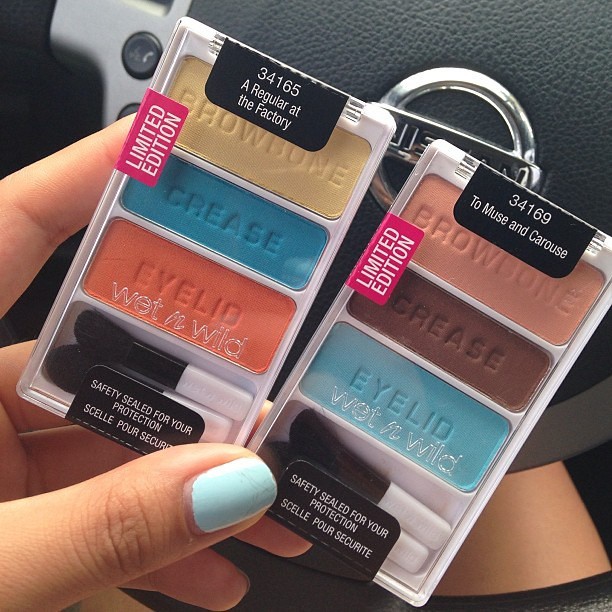In a close-up photograph taken inside a car, a woman with white, bluish sea foam painted fingernails is holding two brand-new eye shadow sets against the steering wheel, which bears the Nissan logo. Each pack contains three distinct eye shadow colors, complete with areas labeled for application: "brow bone" at the top, "crease" in the middle, and "eyelid" at the bottom. The left eye shadow set, titled "34165 A Regular at the Factory," features yellow, blue, and orange hues. The right set, named "34169 To Muse and Carews," includes peach, dark brown, and light blue shades. Both sets prominently display pink stickers indicating they are limited edition, black stickers reading "safety sealed for your protection," and the brand name Wet n Wild in raised plastic. Additionally, each pack comes with two brushes at the bottom.